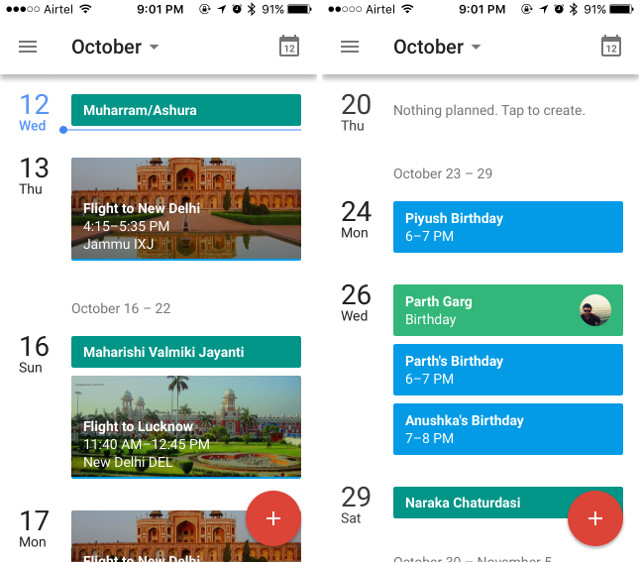A smartphone screenshot displays in detail the user's calendar and upcoming events. In the top right corner, the time reads 9:01 PM with a battery level at 91%. To the left, a hamburger menu is visible, and the top section showcases a drop-down menu labeled "October" accompanied by a calendar icon and a gray divider line beneath it. 

The calendar entry starts with "Wednesday 12th, Muharram Ashura," followed by "Thursday 13th, flight to New Delhi for 15th, 5.35 PM, Jammu IXJ." Below, events from October 16th to 22nd are listed: "Sunday 16th, Maharishi Valmiki Jayanti," and then "Monday 17th," which includes a partial image of a temple, cropped and only partially visible, indicating another "flight to New Delhi."

The adjacent screenshot on the right mentions "23rd day, nothing planned, tap to create," and continues with a header "October 23rd-29th" for the upcoming week.